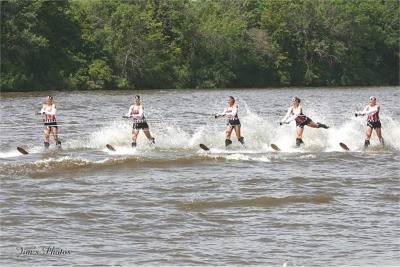This photograph captures a dynamic scene of five women engaged in synchronized water skiing on a lake. Each woman is dressed in a white shirt and black shorts, standing confidently on single slalom skis. They hold onto ropes attached to a boat or watercraft that pulls them in unison across the murky, brownish-gray water. The skis create splashes and waves that add a sense of motion and excitement to the image. Reflective sunlight on the water's surface gives it sporadic hints of light blue and gray. In the far background, a lush line of bright green trees extends down to the water's edge, adding a natural frame to the scene. The bottom left-hand corner of the image features dark gray text that reads "Jim's photos," providing a subtle watermark. The overall impression is one of athleticism and coordination amidst a picturesque lakeside setting.